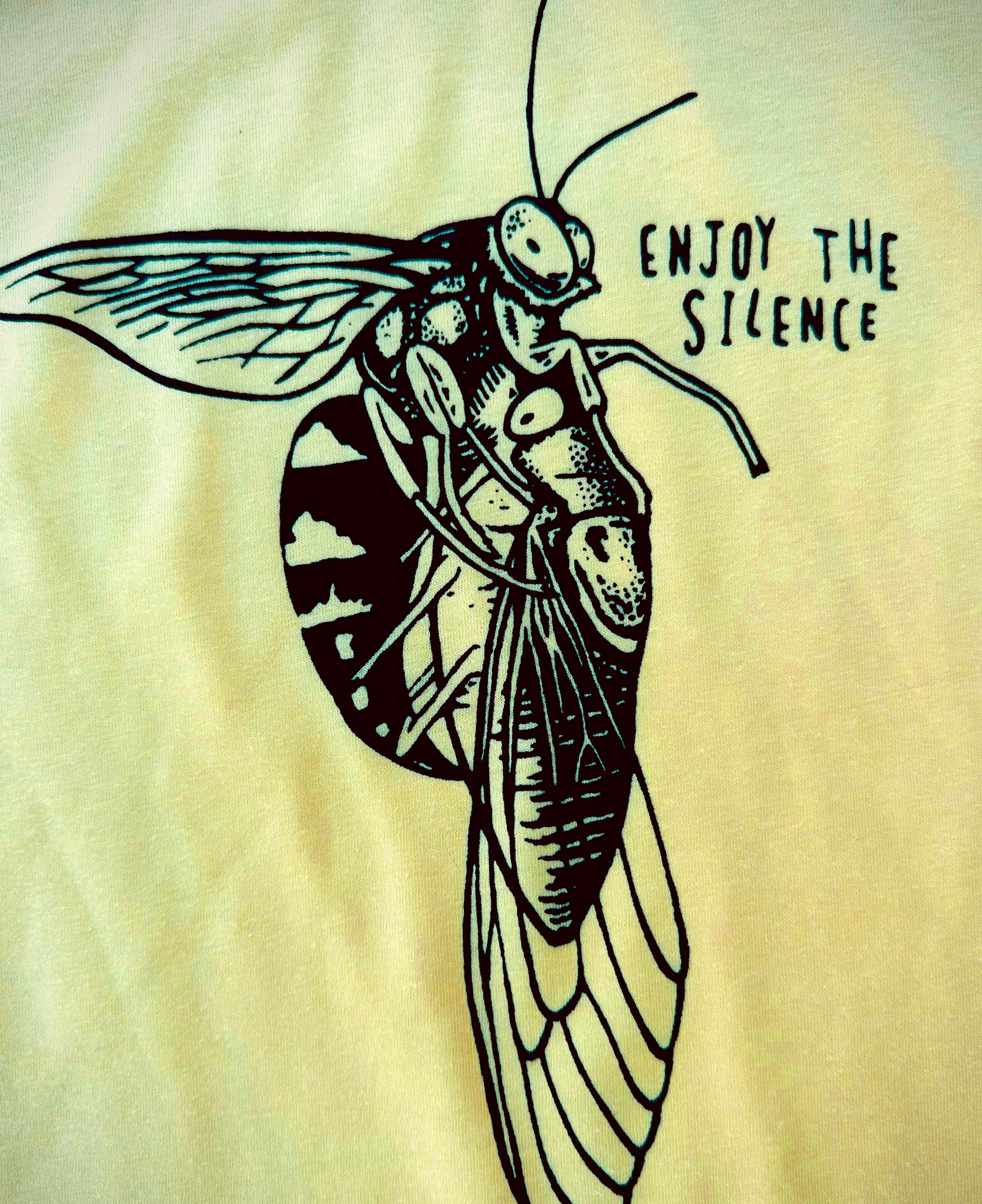This detailed black-and-white illustrated image depicts what appears to be a wasp next to a cocoon, though it’s somewhat ambiguous and could be interpreted as two wasps or a wasp alongside a butterfly emerging from a cocoon. The primary figure, which resembles a wasp, is positioned facing to the right with its wings extending behind it to the left. The wasp seems to wrap its legs around the adjacent cocoon-like structure. This cocoon to the right intriguingly has features that suggest a smiley face and two eyes, adding to the overall mysterious nature of the illustration, with a suggestion of wings emanating from it. 

The backdrop of the image starts off-white, gradually darkening towards the bottom and right, while lightening upwards and to the left, almost transitioning into pure white. There's a slight yellow hue in certain areas, particularly in the lower right-hand corner, which transitions to a greenish tint as it moves upward. Prominently, at the top right corner, the phrase "Enjoy the Silence" is inscribed in black lettering, adding a contemplative touch to the surreal scene. The overall artistic composition is a study in contrasts and visual interest, leaving much to the viewer's interpretation.